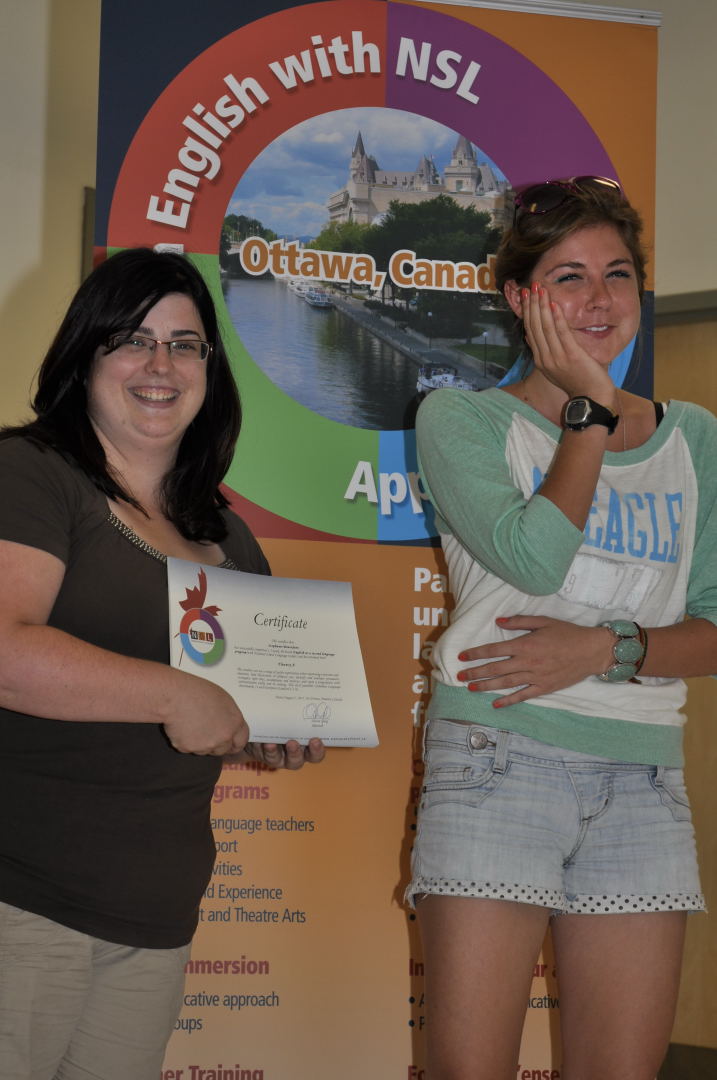This detailed color photograph captures two women standing side by side in a room, showcasing a significant moment. Behind them is a large, vibrant banner with the text "English with NSL" and "Ottawa, Canada" in its center, surrounded by a colorful circular design featuring red, purple, green, and blue segments. Within this circle, there is an illustration of a castle-like building, a lake, a sidewalk, and trees.

The woman on the left has long, straight black hair and is wearing glasses. She is smiling warmly at the camera. She’s dressed in a dark t-shirt and khaki pants, and she’s holding a certificate that has a signature and some paragraphs of writing. The t-shirt appears to be of a brownish or black hue, aligning with different observers' perspectives.

The woman on the right is taller with light brown hair, and she has sunglasses perched on top of her head. She is also smiling, and her right hand rests thoughtfully on her chin while her left hand is positioned around her midsection. She is dressed in a white t-shirt with green, three-quarter length sleeves and blue denim shorts, which are described as having polka-dot patterns from certain angles. She accessorizes with a black watch on her right wrist and a wristband with light green gems.

This photograph effectively captures the joyful atmosphere and the connection between the two women, set against the backdrop of a meaningful and vibrant display.